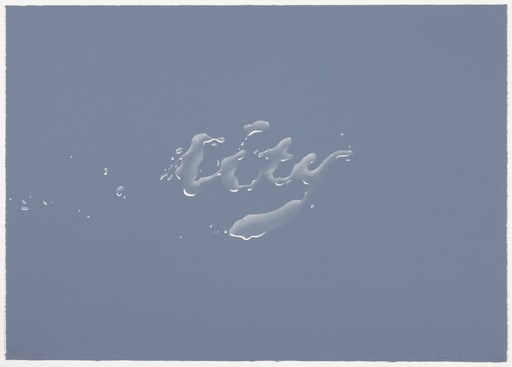The image depicts a digital artwork, almost square but slightly wider than tall, featuring a smooth, medium to dark grayish-blue background. At the center of the composition, the word "city" is spelled out in cursive using dynamic water splashes. The lettering appears shiny, incorporating subtle highlights with varying shades of white and light blue to create a three-dimensional, reflective look. Surrounding the main text, particularly to the left side, are smaller water droplets and bubbles, suggesting the motion and fluidity of the splash, as if the liquid was sprayed from the left. The overall effect is reminiscent of interactive liquid in a commercial, blending elements of both artistic design and science fiction.